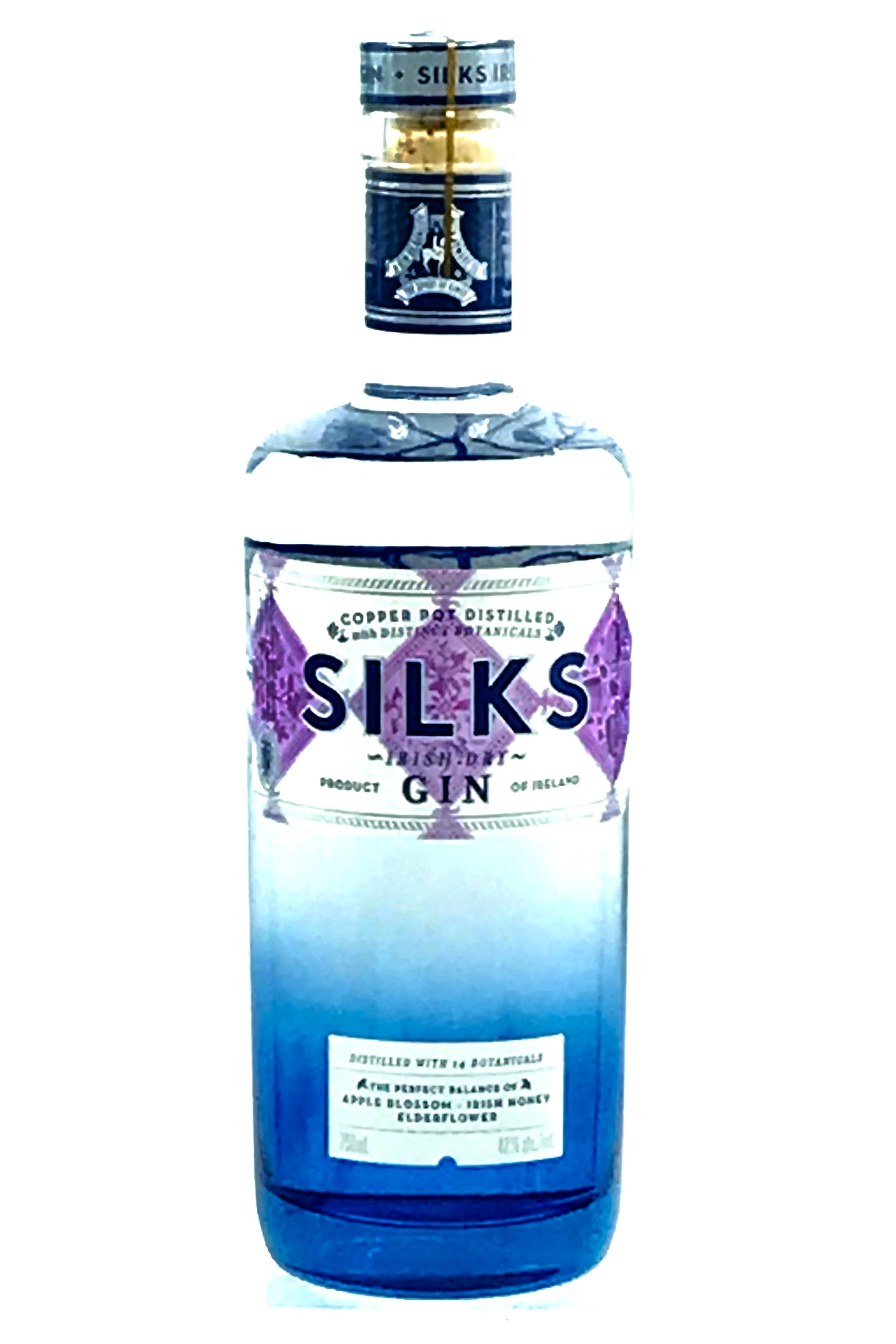The image depicts a glass bottle of Silks Irish Dry Gin, showcasing a gradient design that transitions from a clear top to a deep blue bottom. The bottle features multiple labels with detailed text. At the top, encased in a bluish background, is a cork stopper visibly bearing the brand name "Silks." Below the main label that reads "Silks" in dark blue, it states "Copper Pot Distilled." Further down the bottle, additional text describes it as a "Product of Ireland" and mentions it is "Distilled with 14 botanicals." Another part of the label provides a poetic description: "The perfect balance of two apple blossoms, fresh honey, and elderflower." The bottle is set against a plain white background, enhancing the contrast and visibility of its intricate label details and unique color gradient.